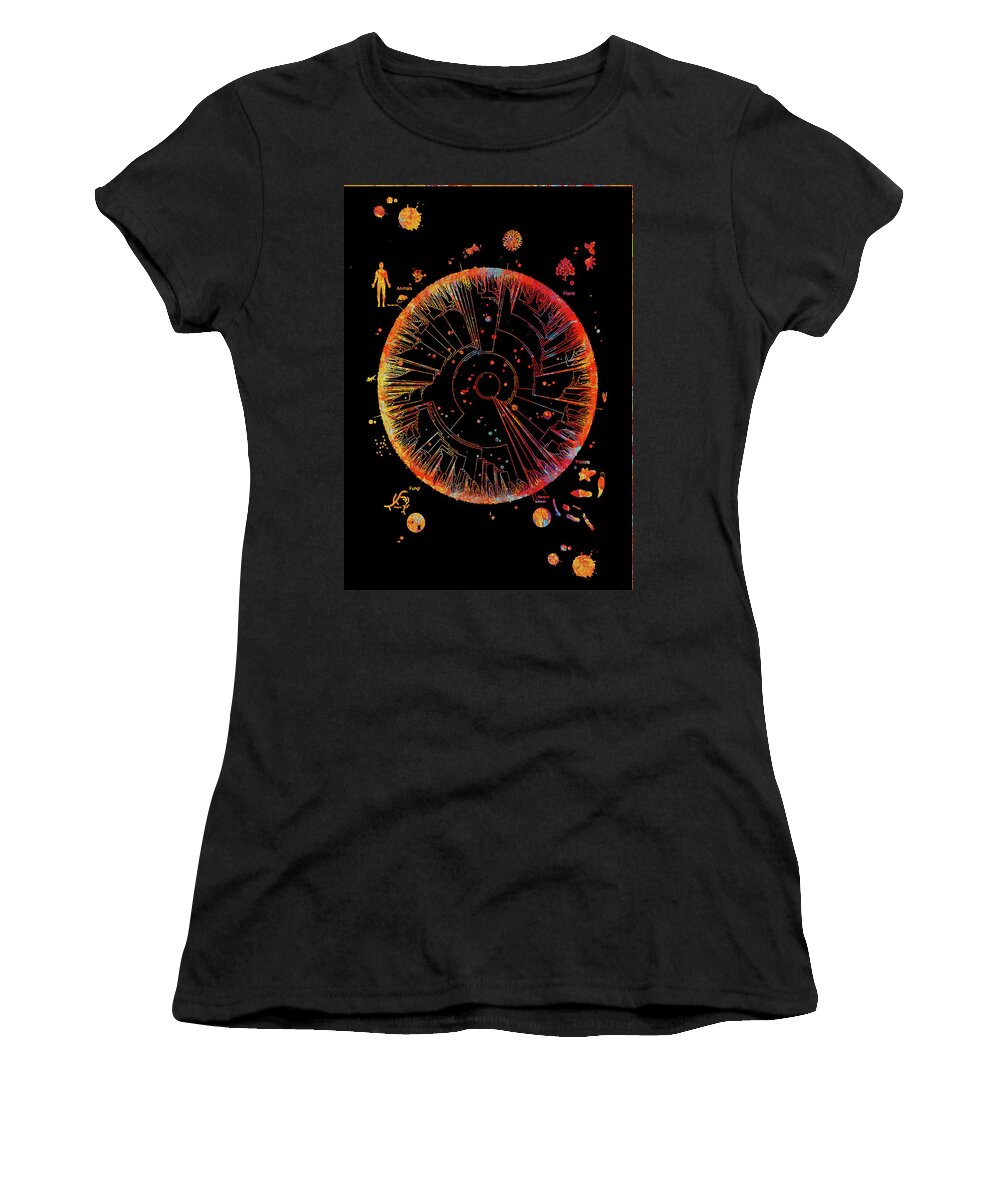This is a product listing photograph of a black women's t-shirt with a ribbed crew neck and slightly capped short sleeves. The t-shirt features a detailed, vibrant design printed on a darker black rectangle positioned in the middle of the chest. The centerpiece of the design is a large cosmic sphere, adorned with a myriad of thin lines and circuits that create the illusion of cosmic circuitry. The sphere is encircled by various shapes, which include intricate representations of life forms, such as human bodies, trees, and fish, potentially illustrating an evolution timeline. Among these shapes, one can distinguish planets, moons, and small metallic-looking orbs that might represent satellites or other celestial objects. The overall color palette includes striking hues of yellow, orange, blue, and pink, giving the design an ethereal, black-light effect. The detailed imagery and absence of text make the t-shirt a captivating piece, perfect for those intrigued by cosmic and evolutionary themes.